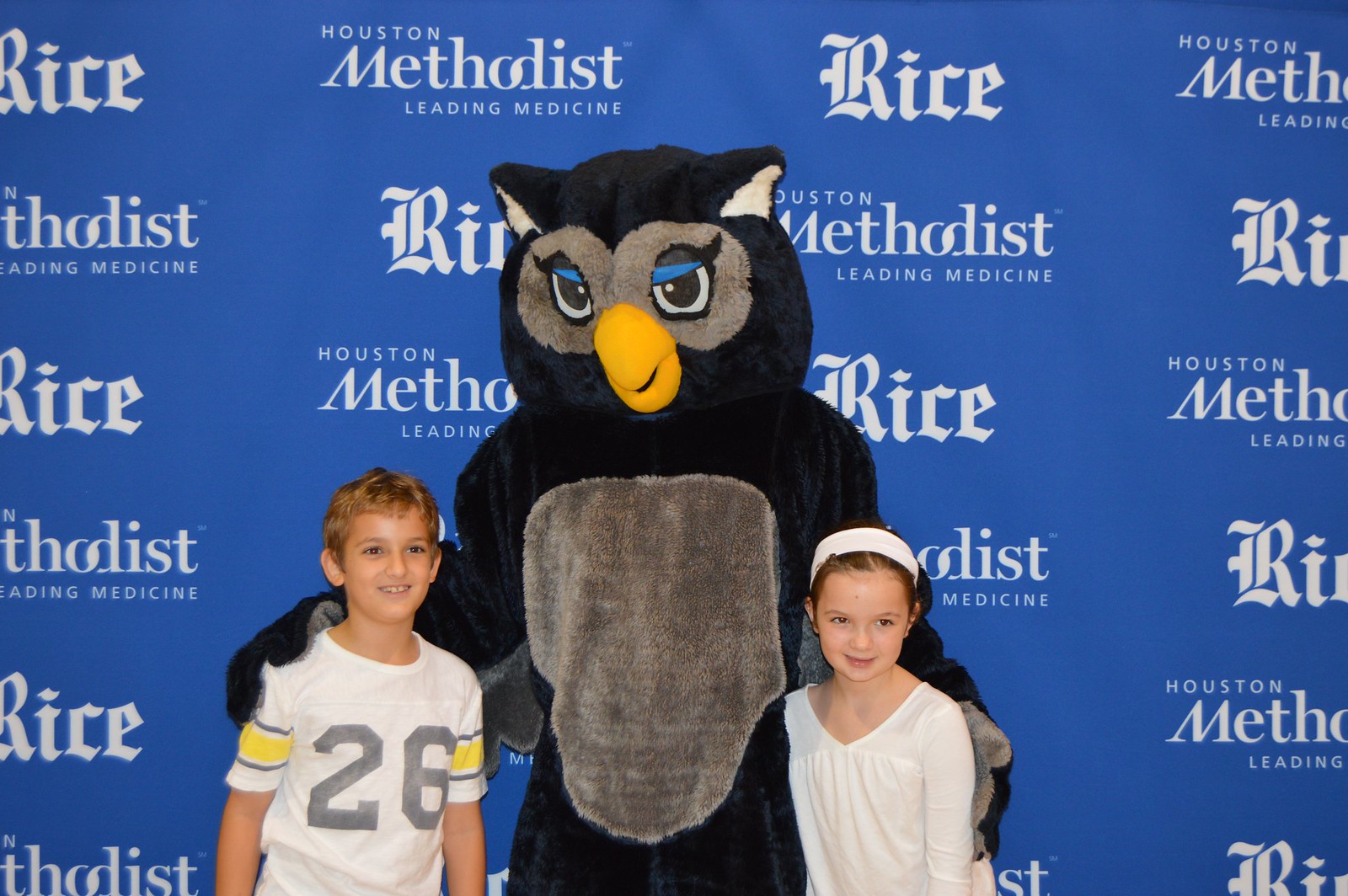In this color landscape photograph, captured at what appears to be a sports event, the central focus is a large owl mascot standing with its arms around two young children, all looking towards the camera. The owl mascot has black feathers, a lighter gray belly, and vibrant details including a yellowish-orange beak and blue eyelids. To the left of the mascot, a boy around 8 to 10 years old, of Caucasian descent, smiles with his mouth open, looking towards the right. He wears a short-sleeve white jersey with yellow bands on the arms and the number 26 in black. On the right, a young girl of similar age, also Caucasian, stands slightly shorter than the boy. She smiles, her hair pulled back and topped with a white bandana, wearing a long-sleeve white V-neck shirt. The backdrop features a blue curtain repeatedly printed with the logos "Houston Methodist Leading Medicine" and "Rice," suggesting institutional sponsorship likely related to a sport or community event. The detailed colors in the image include blue, white, gray, yellow, brown, and tan, emphasizing the lively and engaging atmosphere.